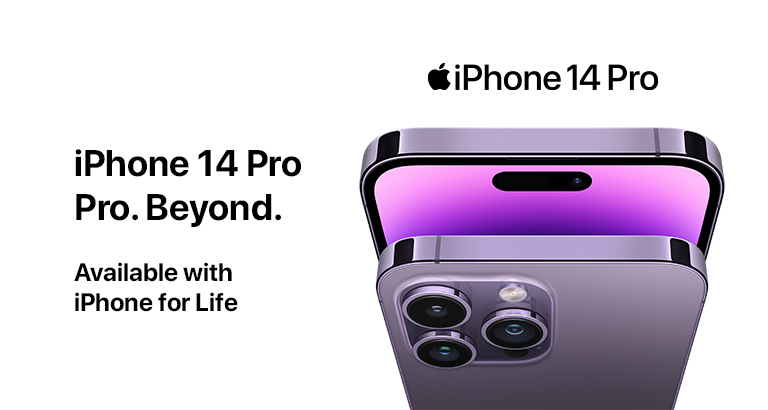Ad Description for the iPhone 14 Pro:

On the left side of the ad, bold black letters prominently display "iPhone 14 Pro." Beneath this, the tagline "Pro. Beyond." captures attention. Just below, in smaller text, it reads "Available with," followed by "iPhone for life" on the next line. 

The right side of the ad features the iconic Apple logo, accompanied by the text "iPhone 14 Pro." Directly under this is a striking image of the iPhone 14 Pro. The phone is depicted from an angle, with its top part pointing upwards and the image tapering narrower toward the bottom, creating a dynamic visual effect. The iPhone is shown in a sleek, shiny silver color with rounded edges that enhance its sophisticated appearance.

The screen of the phone exhibits a gradient purple hue, adding an element of elegance and modernity. At the bottom part of the phone, three camera lenses are visible, signifying its advanced photographic capabilities. Above the camera lens on the right is a small round flash, ensuring excellent photo quality in various lighting conditions.